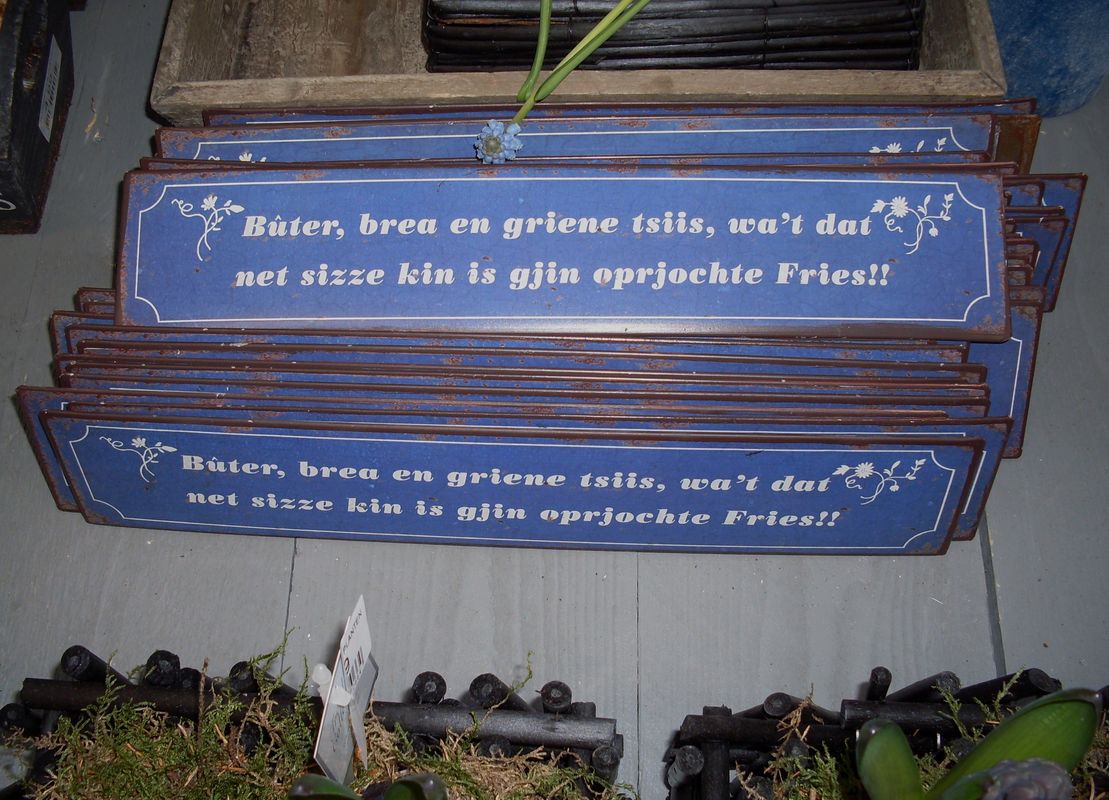The image features a detailed arrangement of objects on a white wooden floor. The most prominent elements are a stack of metal signs, which are blue with rusted edges, white borders, and white text in a foreign language. The signs' text reads: "B U with an upside-down V over the U, T E R comma space B R E A space E N space G R I E N E space T S I I S comma space W A apostrophe T space D A T and the next line N E T space S I Z Z E space K I N space I S space G J I N space O P R J O C H T E space F R I E S!!" The signs seem weathered, indicating they might have been outdoors for a while. They are resting against a rectangular container made of wood or metal bits, possibly the aforementioned wooden crate. This crate has a plant or necklace dangling from the top, adorned with green leaves and a flower with white petals and an orange center. In the lower part of the image, various plants are visible, some displaying green and yellow moss, while others are more leafy and green. Small white decorative flowers are also part of the scene, adding to the rustic and botanical theme of the photograph.